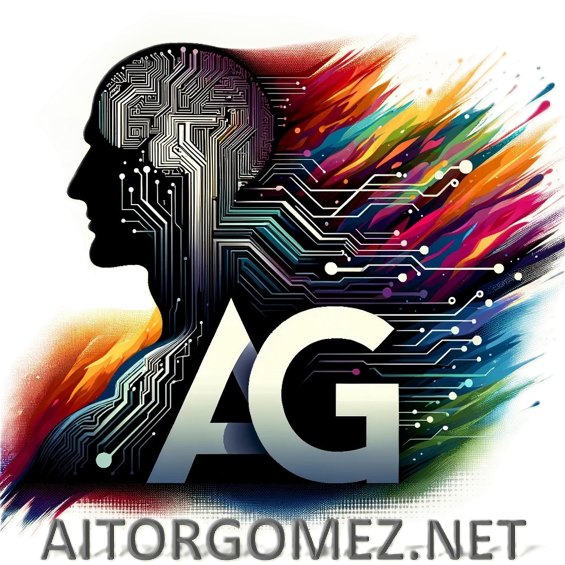This digital graphic art illustration features a dramatic, abstract composition centered around the black silhouette of a bald man in profile, facing left. The man's pronounced nose and chin are silhouetted, creating a stark outline. Within his head, where the brain would be, is a complex white circuit board pattern with notably close-knit lines and circular nodes, evoking the intricate design of a motherboard. This circuit motif extends from his head down through his body and across the image, primarily towards the right side, ending in more circular nodes. 

The background bursts with vivid, flame-like streaks of color, ranging from reds and oranges to blues, greens, purples, and golds, creating a striking contrast against the dark silhouette. These colorful streaks originate from the lower left corner and fan out diagonally across the image, adding a dynamic, almost chaotic energy to the piece.

In the bottom center are two large, overlapping letters "A" and "G", filled with a neutral gradient that transitions from dark at the bottom to light at the top. Beneath these letters, in embossed gray text, is the artist's website, "AitorGomez.net". The overall composition merges elements of technology and vibrant color, resulting in a visually compelling and thought-provoking image.